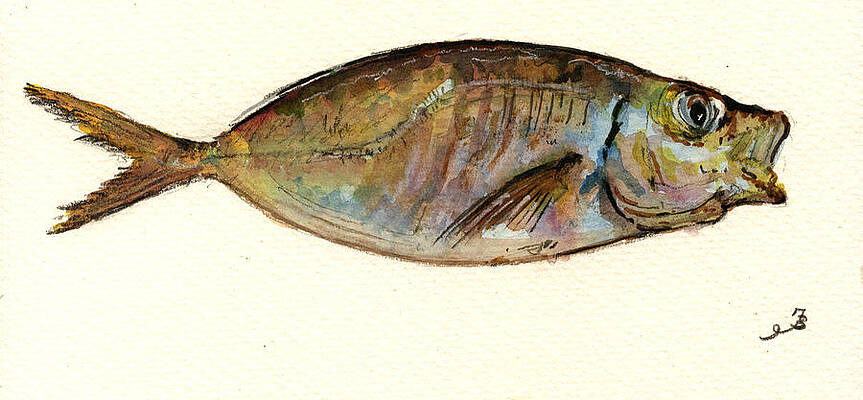In this detailed painting, a fish is prominently featured against a light cream-colored, textured background. The fish is positioned in the top half of the canvas, with its almond-shaped body facing right and its mouth slightly open. The fish, rendered in watercolor, has a striking color gradient that starts with black at the top and transitions through brown, green, purple, and blue hues. The tail, fanning out on the left side of the image, is composed of two thin triangular shapes in brown with yellow accents. The eye has a notable blue haze around it, with additional blue tones extending towards the keels near the bottom side and back of the head. A delicate black pencil signature, possibly consisting of initials and numbers, is present in the bottom right corner of the painting.